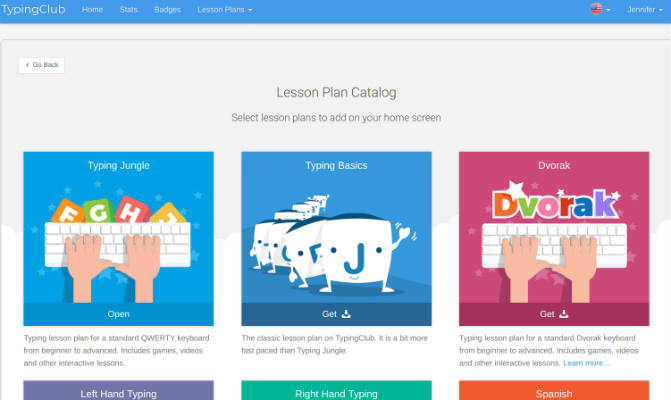This is a screenshot of the TypingClub website, showcasing its colorful and engaging interface. Prominently displayed in the center of the page are three horizontally aligned boxes, each featuring cartoon-like images that include characters with animated square bodies, arms, legs, and letters of the alphabet centered on them. These boxes represent different typing courses: the one on the left is labeled "Typing Jungle," the center box is titled "Typing Basics," and the right box is marked "Dvorak."

At the top left corner of the webpage, the TypingClub logo is displayed, accompanied by a navigation menu with options such as Home, Stats, Badges, and Lesson Plans. On the far right corner at the top, there is a circular icon resembling a user's profile picture with the name "Jennifer" next to it, indicating a logged-in user.

In the center of the page, a prominent heading reads "Lesson Plan Catalog," followed by an instruction: "Select lesson plans to add to your home screen." The page layout and design combine engaging visuals with clearly designated sections for ease of navigation.